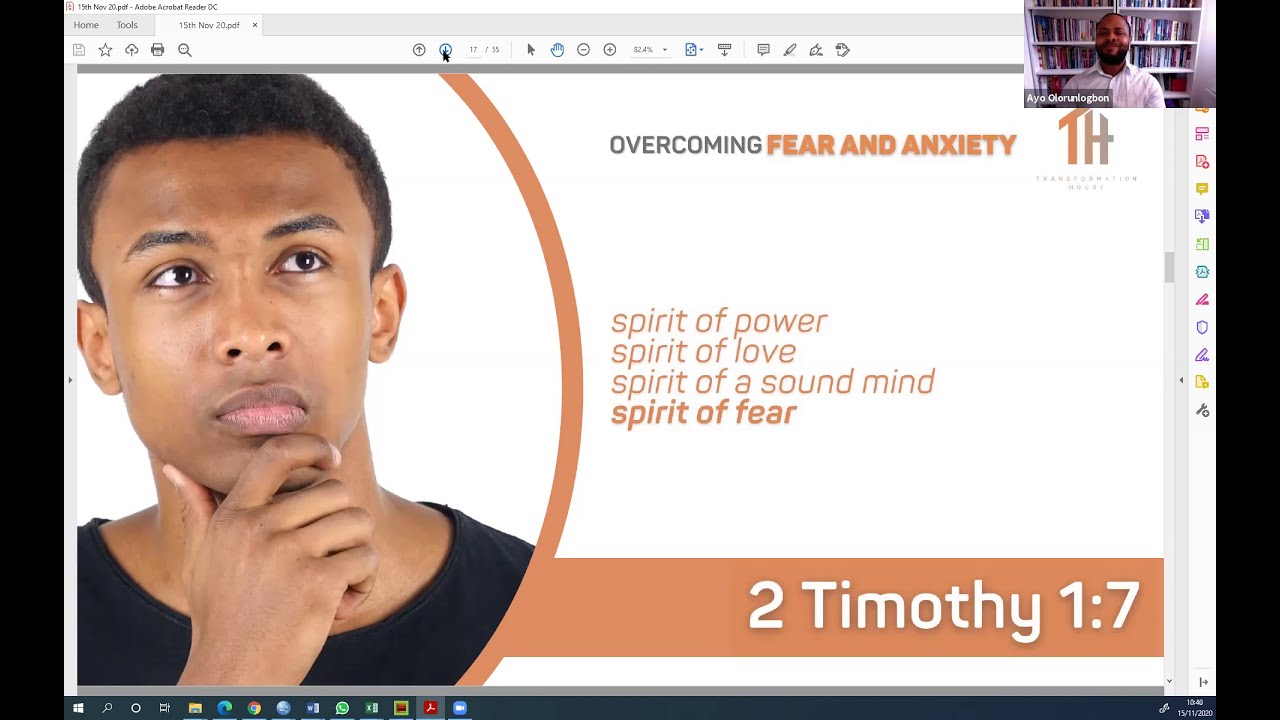The image displays a screenshot of a computer screen running on Windows, evident by the taskbar with multiple icons at the bottom. The main focus of the screenshot is a presentation slide, presumably displayed using Acrobat Reader. On this slide, there is a high-quality image of an African-American man with short black hair, a black beard, and a mustache. The man, Ayo Olorunlogbon, is wearing a black shirt and is thoughtfully resting his hand on his chin.

To the right of the image, the slide's title reads in all capital letters "OVERCOMING FEAR AND ANXIETY," with "overcoming" in gray font and "fear and anxiety" in a brownish-orange font. Below the title, four lines of text list: "Spirit of power," "Spirit of love," "Spirit of a sound mind," and "Spirit of fear." At the bottom of this section, in white font, is the scripture reference "2 Timothy 1:7."

In the upper right corner of the presentation slide, there is a video feed of the presenter, who appears to be the same African-American man from the slide. He is dressed in a white collared button-up shirt. Behind him, a large white bookshelf filled with numerous books is visible, adding context to his professional or academic environment.